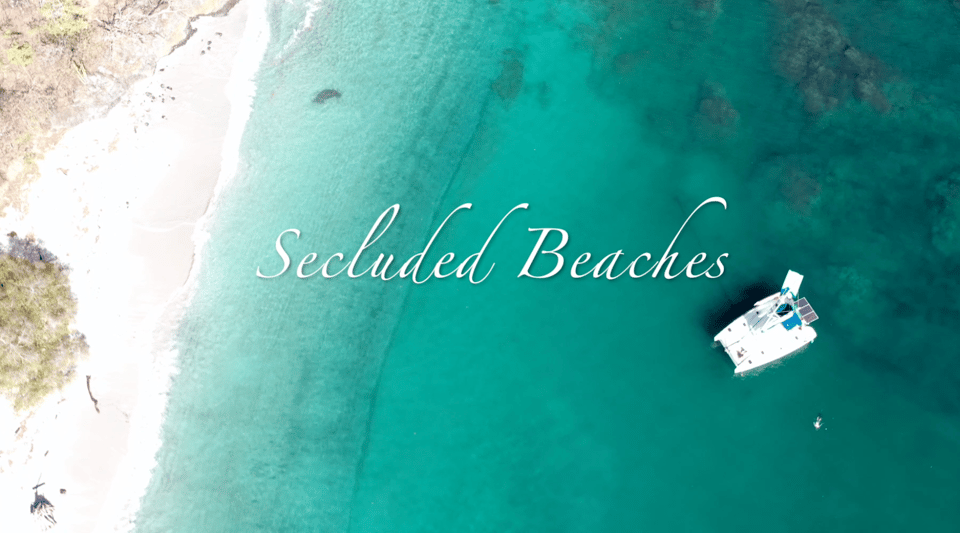This aerial photograph captures a serene, secluded beach flanked by a clear, turquoise-blue ocean. On the left side, occupying about 25% of the image, is a white sand beach adorned with various sea flora in shades of green and brown. Atop the beach, part of a tree or possibly some bushes is visible. The remaining 75% of the image showcases the pristine ocean, where the water is so clear you can slightly see through it to the seabed below. In the lower right corner, a large white yacht with blue accents is partially visible. Centered in the water, the phrase "secluded beaches" is elegantly displayed in white text, seamlessly blending into the tranquil scene.